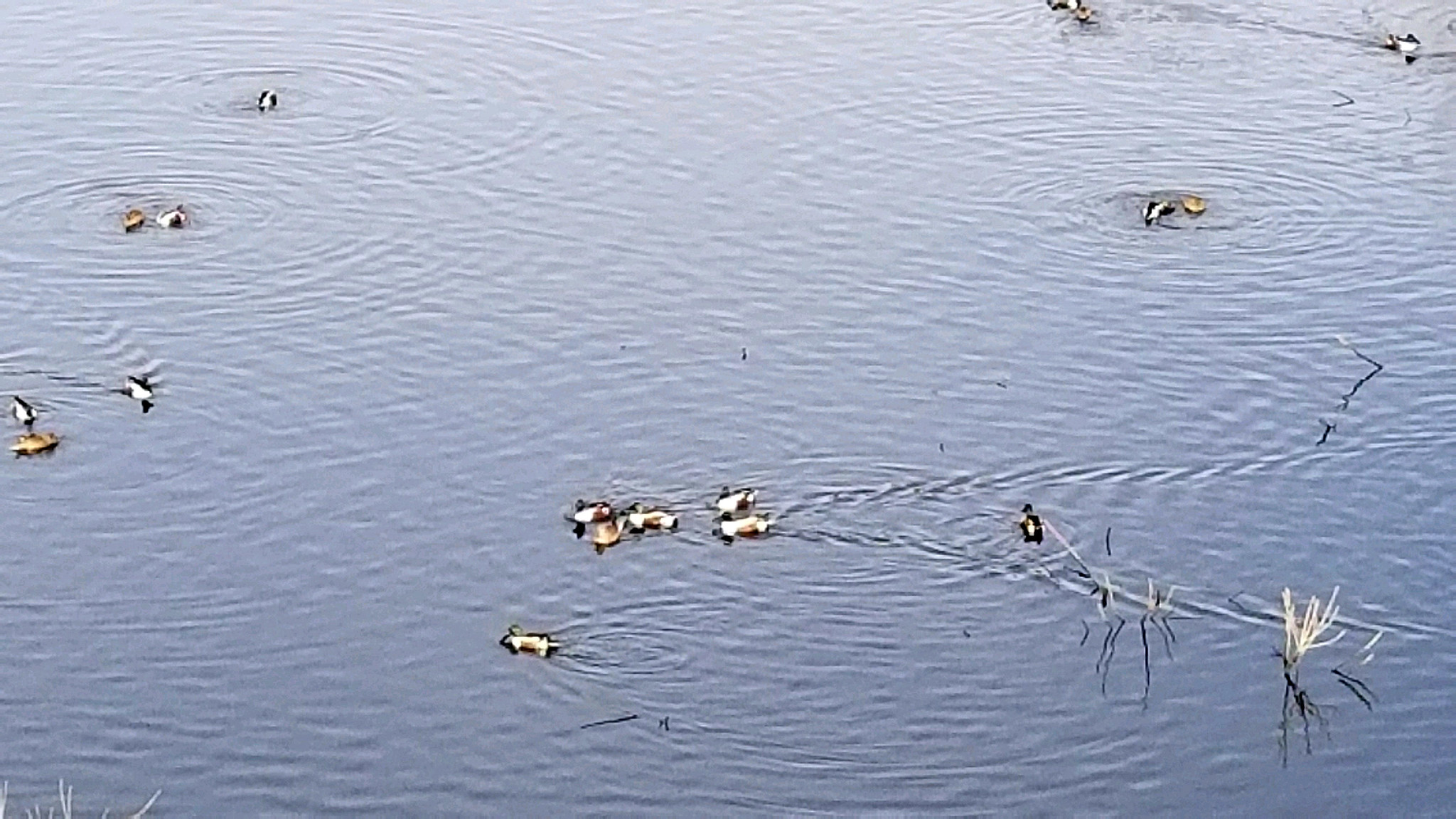Aerial photograph of a serene, grey-blue lake covered with gentle ripples created by numerous ducks gracefully gliding across the water. In the center of the image, a group of five ducks swims forward, producing distinct V-shaped ripples behind them. Scattered across the lake are additional groups of ducks: six in the middle, five spread to the left, and another five to the right, totaling sixteen ducks. The ducks display varying color patterns including brown heads, some with white bodies and brown feathers, and others with yellowish-brown tones. In the lower right corner and along the sides of the image, white reeds poke through the water, adding an element of texture and natural detail. The overall scene evokes a peaceful, gently bustling aquatic habitat.